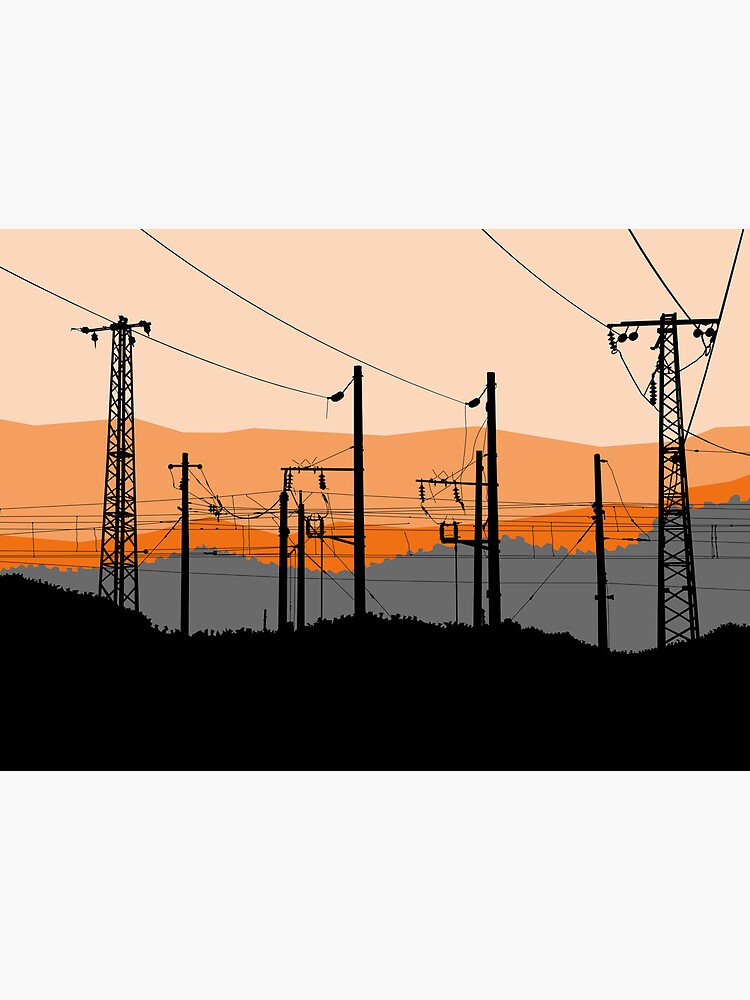The image depicts a digital art piece of a landscape dominated by numerous power towers and crisscrossing electric cables extending across a vast field. The scene unfolds under a striking sky transitioning from pink and orange hues near the horizon to a gray tone higher above, suggesting either early morning or sunset. Stretching into the horizon, the power lines and utility poles stand tall and interconnected, with some wooden telephone poles interspersed, all amidst grassy terrain. The landscape includes a series of mountains or hills, which change in color from dark and light orange to black as they recede into the background, enhancing the depth of the composition. The meticulous detailing of the interconnected power infrastructure contrasted against the gradient sky highlights the intersection of human engineering and natural beauty.